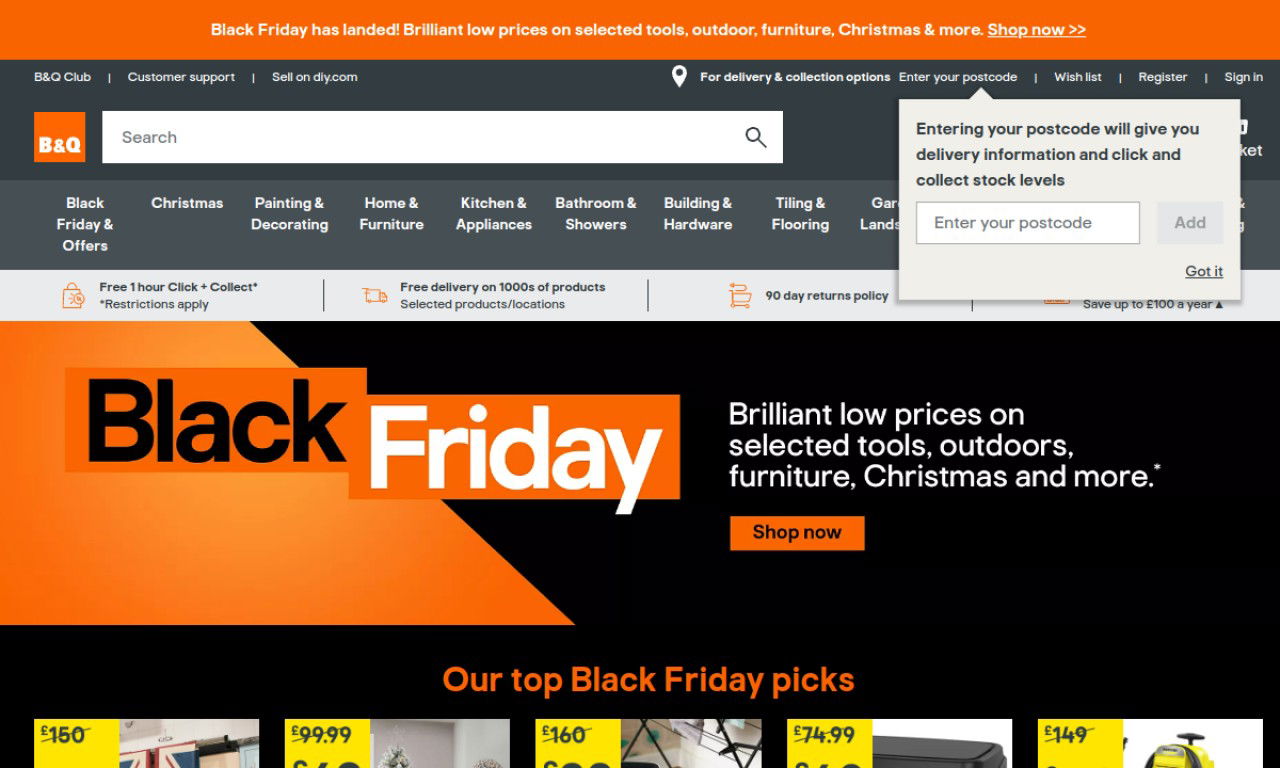This screenshot is from a computer displaying a promotional webpage for B&Q Club. The banner prominently advertises significant savings, offering up to £250 off on selected garden furniture, barbecues, and spa products, encouraging users to "Shop Now." The interface features intuitive navigation with categories such as Building & Hardware, Bathroom & Showers, and Kitchen & Appliances, enabling users to easily locate their desired sections. A noteworthy inclusion is a large search box for quick access to specific items. Additionally, a useful input box prompts users to enter their postcode, providing relevant delivery information and local stock availability for click and collect services. Other highlights include a 90-day return policy, free delivery options, and a vast selection of products. The webpage also boasts 50% off on selected outdoor living items during the summer clearance event, with immediate access to the sale through another "Shop Now" link. A free one-hour click and collect service is available, although certain restrictions apply. Some offers appear to be cut off at the bottom of the page, leaving a sense of anticipation for additional deals.